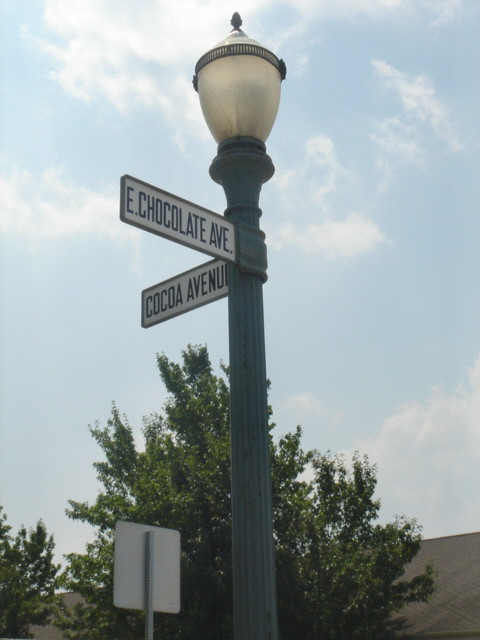The image captures a vibrant scene under a clear blue sky filled with white, fluffy clouds. At the top of the frame, lush green leaves contrast beautifully against the sky. In the foreground stands a metal pole tipped with a glass lantern, adding a touch of vintage charm to the setting.

Towards the left side of the image, a white rectangle, possibly a sign, is mounted on a gray structure, which might be a rooftop with a slight slope. This structure is supported by a metal pole with four noticeable holes in it. Adding to the urban landscape, a white square sign is prominently displayed, indicating the intersection of "BlackTex East" and "Chocolate Avenue." Perpendicular to this is another sign pointing towards "Cocoa Avenue," providing a sense of direction and place within the image.